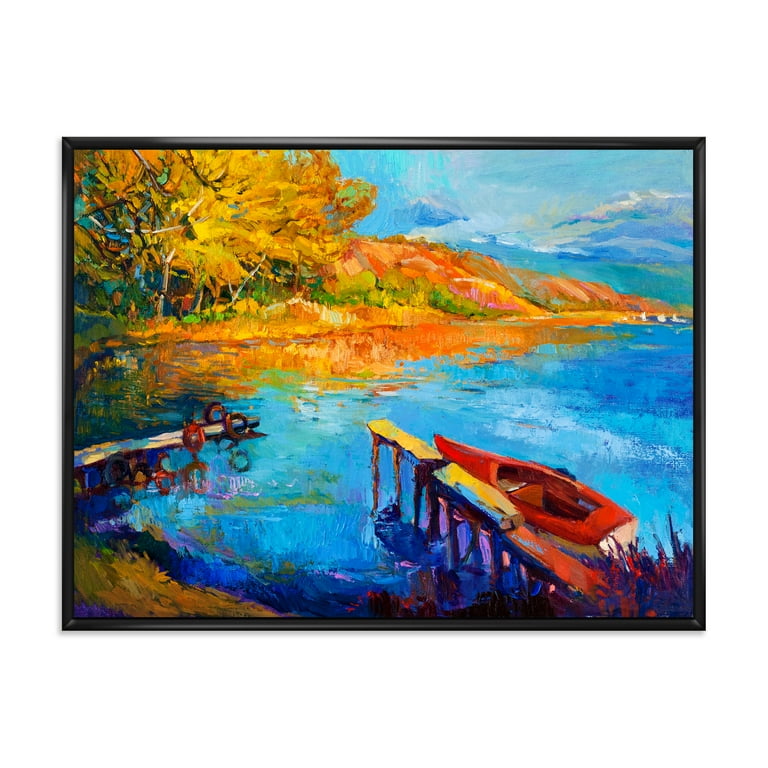This watercolor painting depicts a serene nature setting at the outer coast of a crystal blue lake. In the right foreground, a small red and white boat is tied to a slightly rickety, narrow wooden dock. To the left, another dock features tires and flotation devices, including inner tubes and a life preserver. The lake, with its varying shades of blue, beautifully reflects the surrounding landscape and sky. The backdrop showcases hills or rock formations in autumnal hues of browns, greens, yellows, and touches of orange, mirroring down into the water. Tall trees, their foliage reflecting the same autumn palette, frame the scene. Above, a sky of various shades of blue with puffy white clouds adds a tranquil touch, also echoed in the water's reflection.